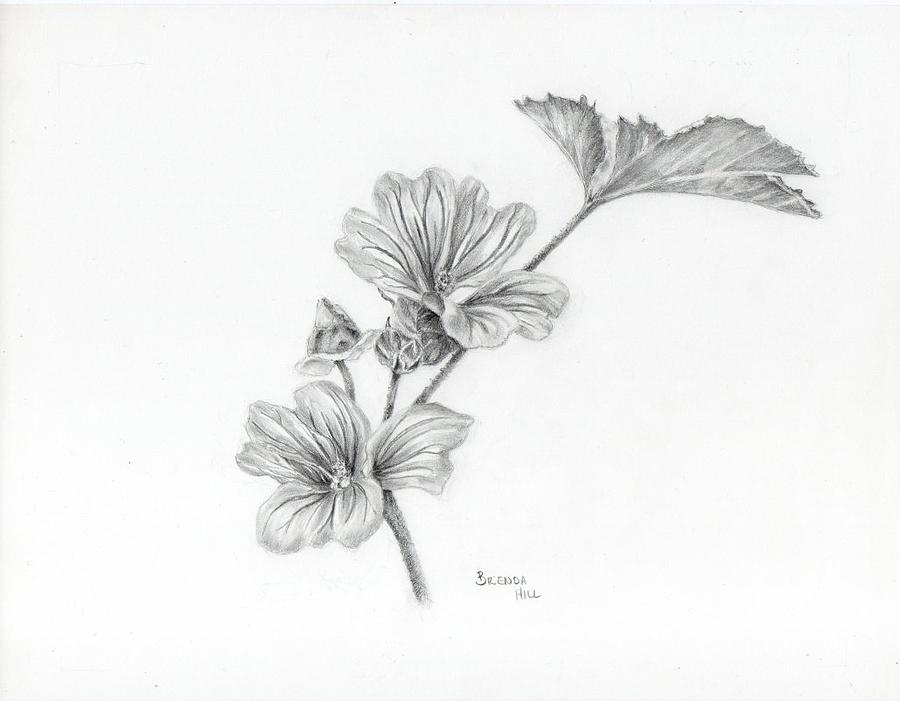This image features a highly detailed, hand-drawn pencil sketch on a white, perhaps slightly off-white, piece of paper. The central focus is a plant with an intricate arrangement of branches, flowers, and leaves. The primary stem emerges from the bottom of the paper, branching out into two smaller stems with small buds, and a third, larger branch extending to the right. This larger branch showcases a prominent flower with many petals, while leaves with visible veins adorn the top. Two flowers have fully blossomed, displaying their delicate petals, while other buds remain unopened. At the bottom of the drawing, to the right of the main stem, the artist's name "Brenda Hill" is clearly inscribed, indicating the creator of this beautiful sketch.